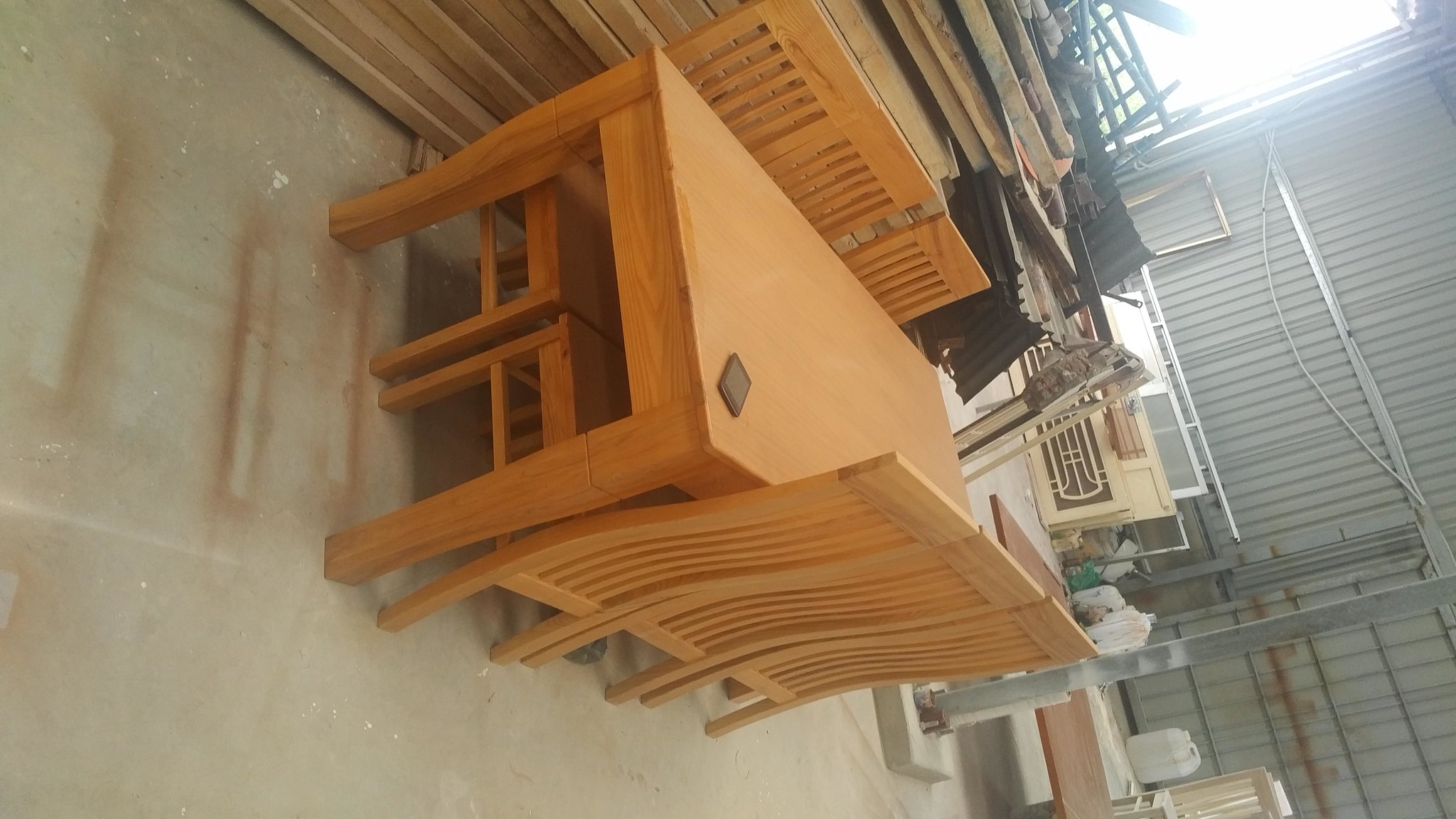This color photograph, though taken at an odd and disorienting angle, captures a wooden table flanked by six matching chairs situated in what resembles an industrial warehouse or possibly an artist's studio. The table, composed of light brown wood, rests on a dirty cement floor. The chairs, three aligned on each side and none at the table ends, feature long backs with wavy patterns and vertical slats, tightly arranged. A black smartphone lies at an angle in the lower right corner of the table. Behind the table, various pieces of lumber are stacked, and a door rests sideways against a metal wall that defines the warehouse background. Additionally, a large metal wall with an opening at the upper right corner is visible, along with a plastic jug sitting at the bottom right of the image. Bright light streams in through an open window, further illuminating the scene.